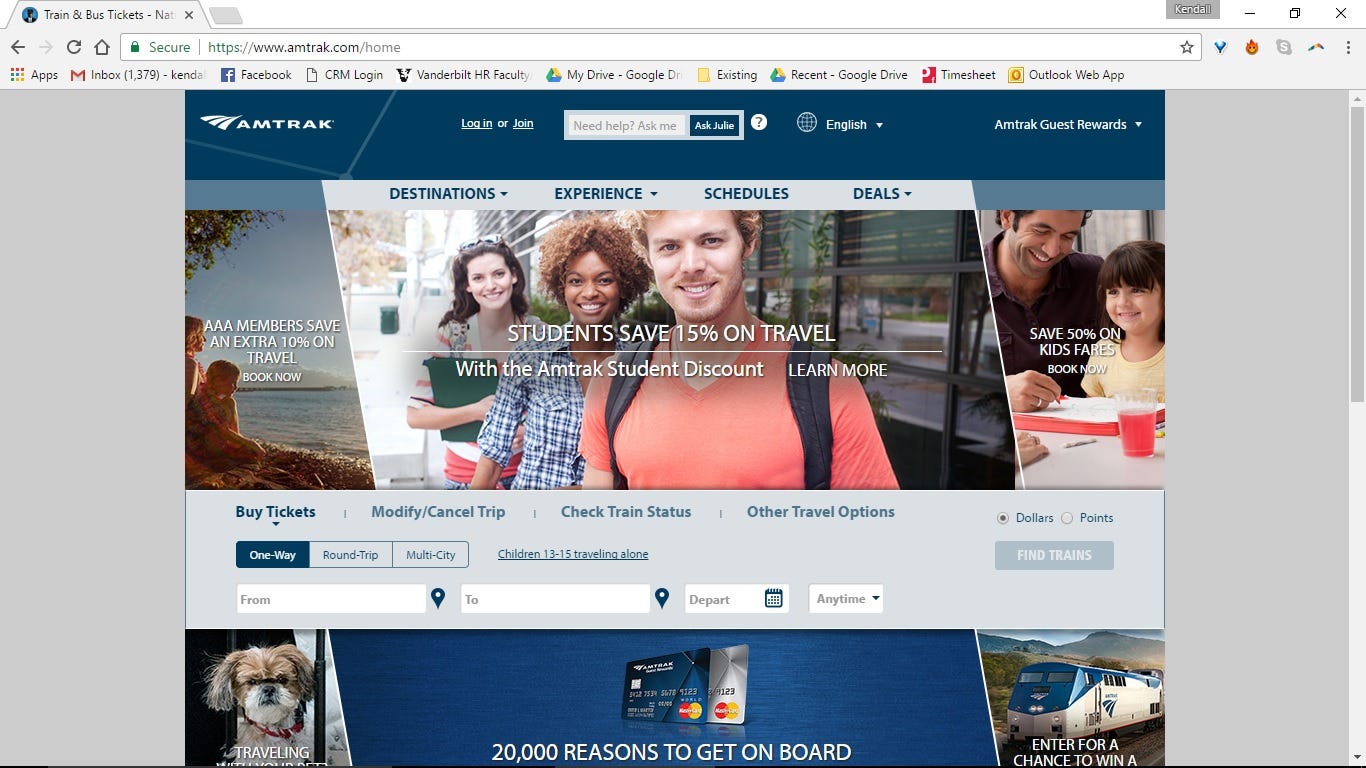This is a detailed screenshot from the Amtrak website. The URL at the top reads: https://www.amtrak.com, home. At the upper section of the page, there are navigation options including "Amtrak," "Log In or Join," "Need Help? Ask Julie," "English," "Amtrak Guest Rewards," "Destinations," "Experience," "Schedules," and "Deals."

On the left side of the webpage, there is a photograph featuring a woman and a child sitting by a shore, gazing at a body of water. A promotional banner over this image reads, "AAA members save an extra 10% on travel. Book now."

Next to this, there is a second image showing a group of three individuals. In the back, a fair-skinned woman with long dark hair has a pair of sunglasses resting on top of her head and holds a green binder under her arm. In the middle stands a dark-skinned woman with short curly hair, smiling directly at the camera. She is wearing a plaid button-down shirt with the sleeves rolled up. At the front, a young man with wavy short blonde hair, a mustache, and a slight beard completes the trio. The caption over this image reads, "Students save 15% on travel with the Amtrak student discount. Learn more."

The final image portrays a man looking down with a big smile. Next to him, a little girl with short dark hair sits beside him. The accompanying text states, "Save 50% on kids' fares. Book now."

Beneath these images, the website offers various options such as "Buy Tickets," "Modify," "Cancel Trip," "Check Train Status," "Other Travel Options," with selectable buttons for "Dollars," "Points," "Find Trains," "One-Way," "Round-Trip," "Multi-City," "Children 13 to 15 Traveling Alone," "From," "To," and "Depart Anytime."

Additionally, there is an option for "Traveling with your pet" below an image of a small dog. Another promotion reads, "20,000 reasons to get on board," accompanied by an image of two Amtrak-branded MasterCard credit cards. At the bottom of the screenshot, partially visible text beneath an image of a blue and white Amtrak train invites users to "Enter for a chance to win A." The rest of the text is cut off at the lower edge of the image.